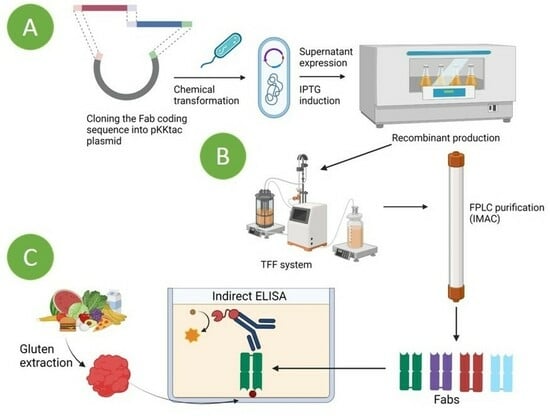This large square infographic with a white background depicts a detailed flowchart utilizing colorful drawings and lab equipment images, organized into three areas labeled A, B, and C. 

In area A, the process begins with the text "cloning the FAB coding sequence into PKK-TAC plasmid," followed by an arrow indicating "chemical transformation." Next, there's imagery resembling a little sperm cell and another arrow leading to "supernatant expression, IPTG induction." This is adjacent to an oven-like device labeled "recombinant production," followed by an arrow pointing rightward towards "FPLC purification, IMAC," and ultimately downward to multi-colored strips labeled "FABs."

Area B appears to centralize around an indirect ELISA (E-L-I-S-A) process, with a box labeled "Indirect ELISA" positioned in the lower mid-left section.

Area C focuses on "gluten extraction," depicted with graphical images of fruits and vegetables. There's an arrow pointing from these food items towards a small red blob, eventually directing towards the "Indirect ELISA" box.

The image also features various arrows, lines (some dotted), and lab equipment illustrations creating a comprehensive visual guide of the described molecular biology procedures.